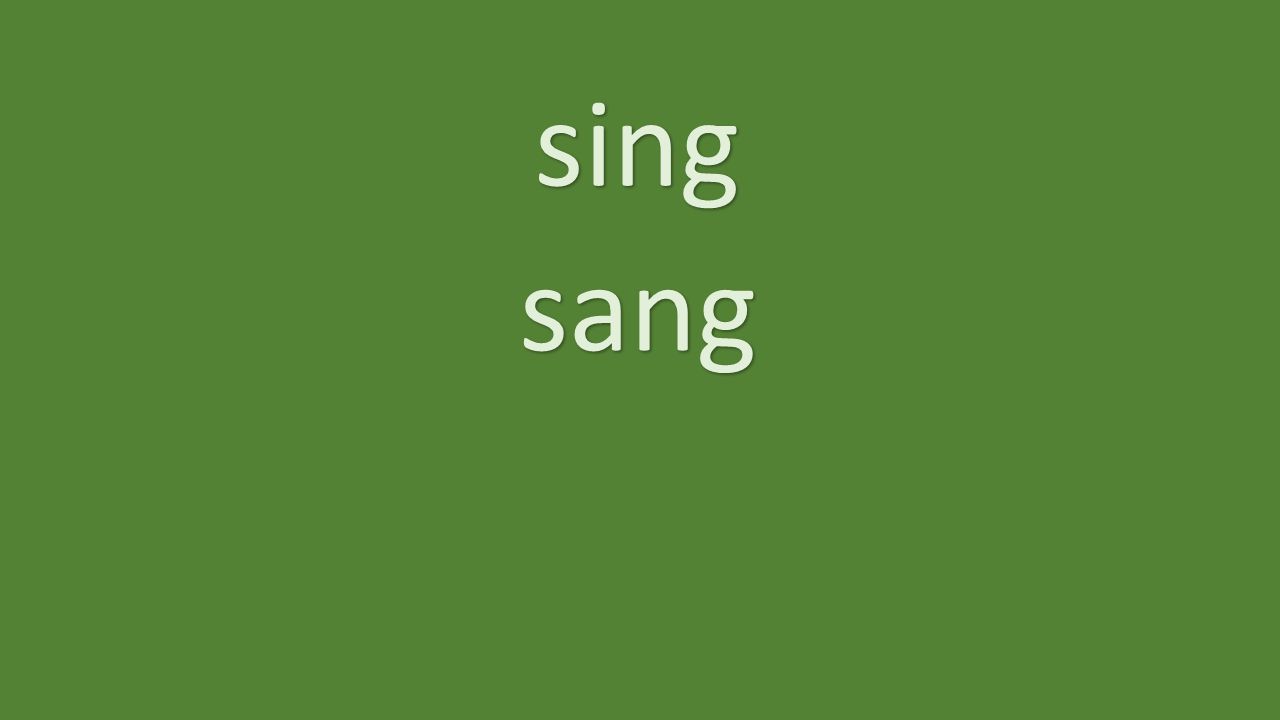The image features a simple design with a solid green rectangular background, where the height is shorter than the width. Near the top middle part of this green rectangle are two words written in lowercase, non-cursive, white letters. The first word, "sing," is positioned slightly above the word "sang." Both words are situated towards the top center of the image. The green background color might be interpreted as a hunter green or forest green. The image has a minimalistic look and could possibly be part of an educational slide about vocabulary or pronunciation, emphasizing the words "sing" and "sang." There are no other objects or elements present in the image.